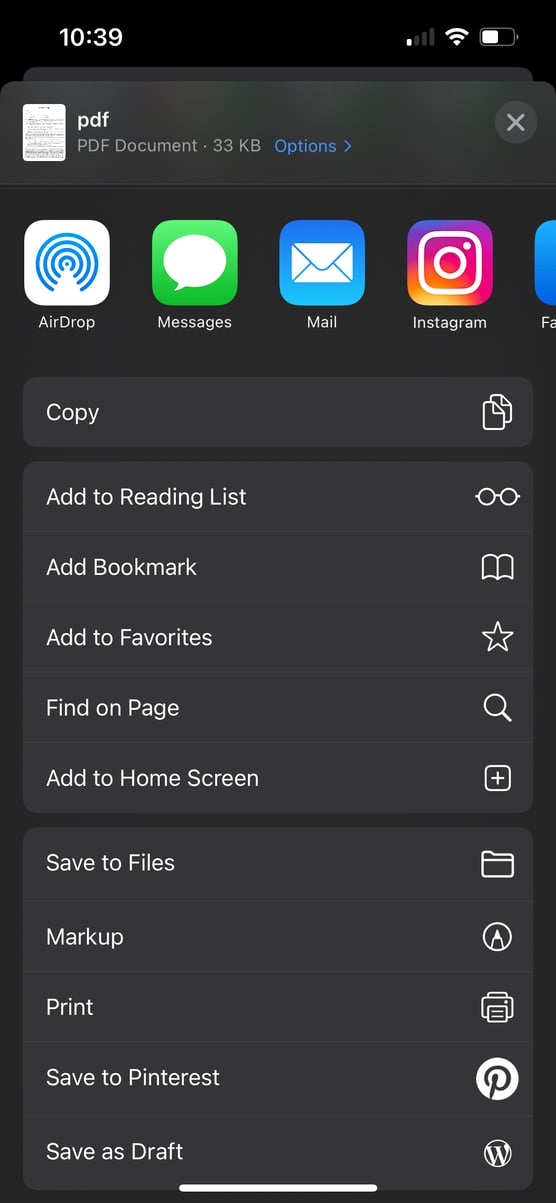The image features a device with a black background and several white icons at the top, indicating the time (10:39), Wi-Fi signal, network strength, and battery level. Below these icons, there is a blue-highlighted pop-up notification at the bottom of the screen that reads "PDF, PDF document 33 KB," accompanied by a blue button labeled "Option" and a white "X" on the right side for closing the pop-up.

Directly beneath the pop-up, there is a horizontal row of application icons: 
1. **Dropbox**: A blue and white icon showing an open box.
2. **Messages**: A green and white speech bubble icon.
3. **Mail**: A blue and white envelope icon.
4. **Instagram**: A gradient purple and white camera icon.

At the bottom of the device screen, there is a menu with several listed options in a vertical formation, each with corresponding white icons to their right:
1. **Copy**
2. **Add to Reading List** with a star icon.
3. **Add Bookmark** with a book icon.
4. **Add to Favourites** with a star icon.
5. **Find on Page** with a search box icon.
6. **Add to Home Screen** with a plus sign icon.
7. **Save to Files** with a file icon.
8. **Mark Up** with a pen icon.
9. **Print** with a printer icon.
10. **Save to Pinterest** with the Pinterest logo.
11. **Save to Draft** with a WordPress icon.

The overall layout is organized and detailed, providing a clear overview of the device's current status, available actions, and accessible applications.